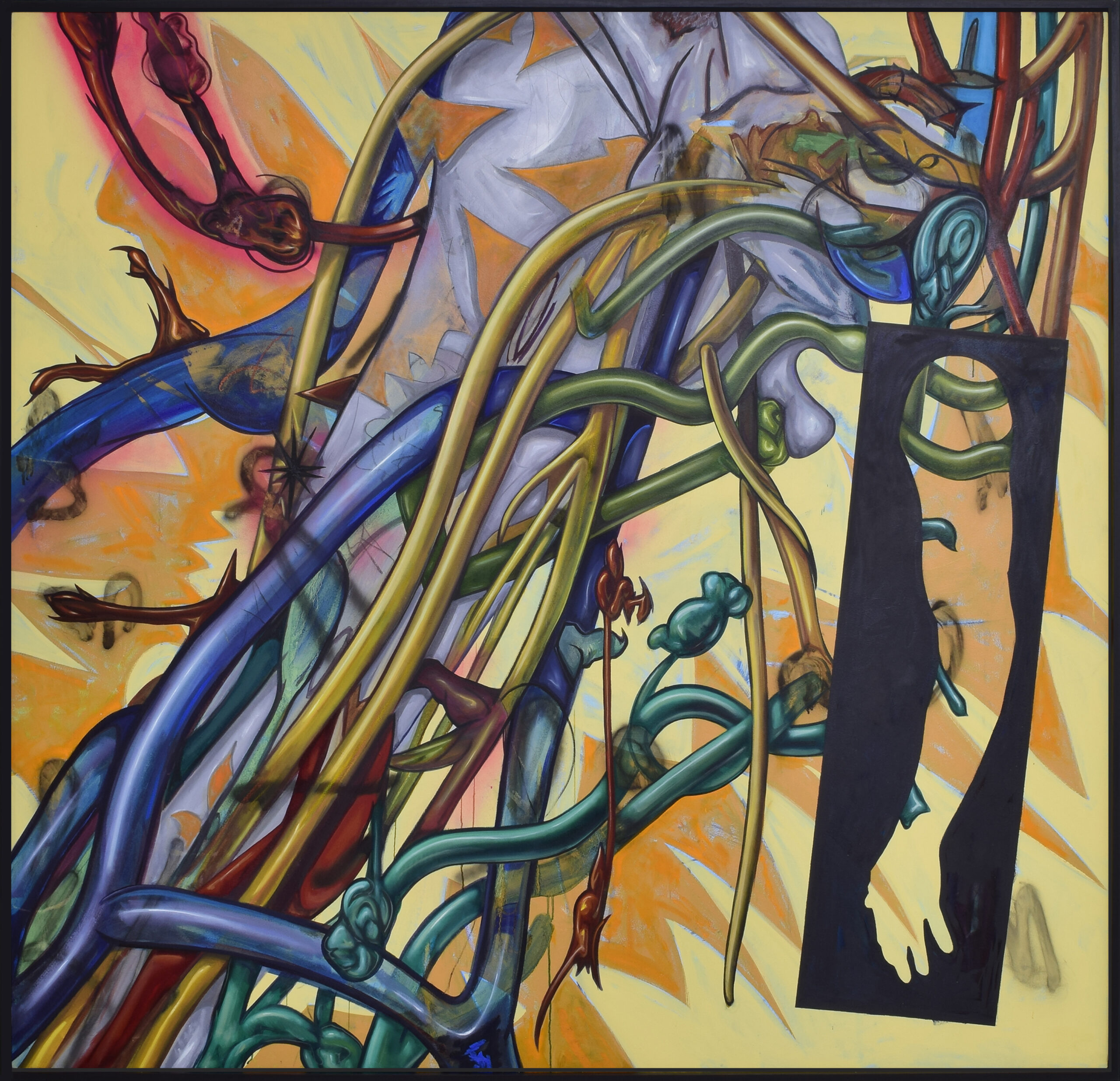This abstract painting features a vibrant palette of yellows, oranges, reds, blues, greens, and blacks. The background is predominantly a pale yellow adorned with sporadic orange zigzags. On the right side of the image, a striking black square holds a cutout silhouette of a human arm, extending from the shoulder to the fingertips, allowing a glimpse of the abstract design behind it.

Dominating the center and spreading from the bottom left to the top center is a large, vine-like purple cylinder decorated with orange triangles. Accompanying this purple vine are a multitude of thinner vines in various colors—yellow, blue, red, and teal—all intertwining and stretching across the canvas. From the top left corner, a magenta vine splits into two, merges back into one, and then converges with the thick purple vine. The top right is a chaotic entanglement of colorful vines, adding to the dynamic complexity of the artwork.

Scattered across the scene are bent, flexible cylinders and several jagged, pointed shapes with curvy edges and occasional bumps and knots, contributing to the painting’s sleek yet indefinably abstract style. In the upper right corner, colored tubes in brown, green, and red descend, with a red organ-like design extending from the left tubing, intertwining with the central purple mass accompanied by additional yellow, blue, and red tubing that twirls throughout the image.